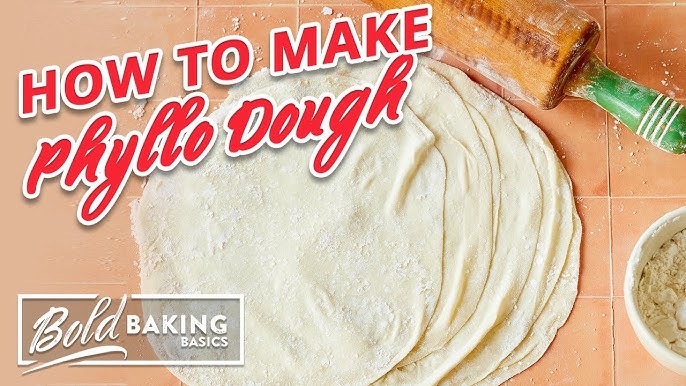This is a full-color, horizontal photograph that appears to be the cover of a book or the first page of a web page, potentially a blog post or Pinterest thumbnail. The title, "How to Make Phyllo Dough," is prominently displayed in bright red text with a white border, situated in the upper left-hand corner. Below the title, a series of thin, round phyllo dough sheets are visibly laid out, overlapping slightly towards the left, with at least six sheets discernible. The background surface is a rust terracotta-colored tile, sprinkled with flour. In the upper right-hand corner, a rolling pin with a green handle rests on the surface. The lower right-hand corner of the image features half of a bowl containing flour. Additionally, in the lower left-hand corner, there is a white rectangle with the text "Bold Baking Basics" written in cursive script and block letters, emphasizing the modern and instructional theme of the image.